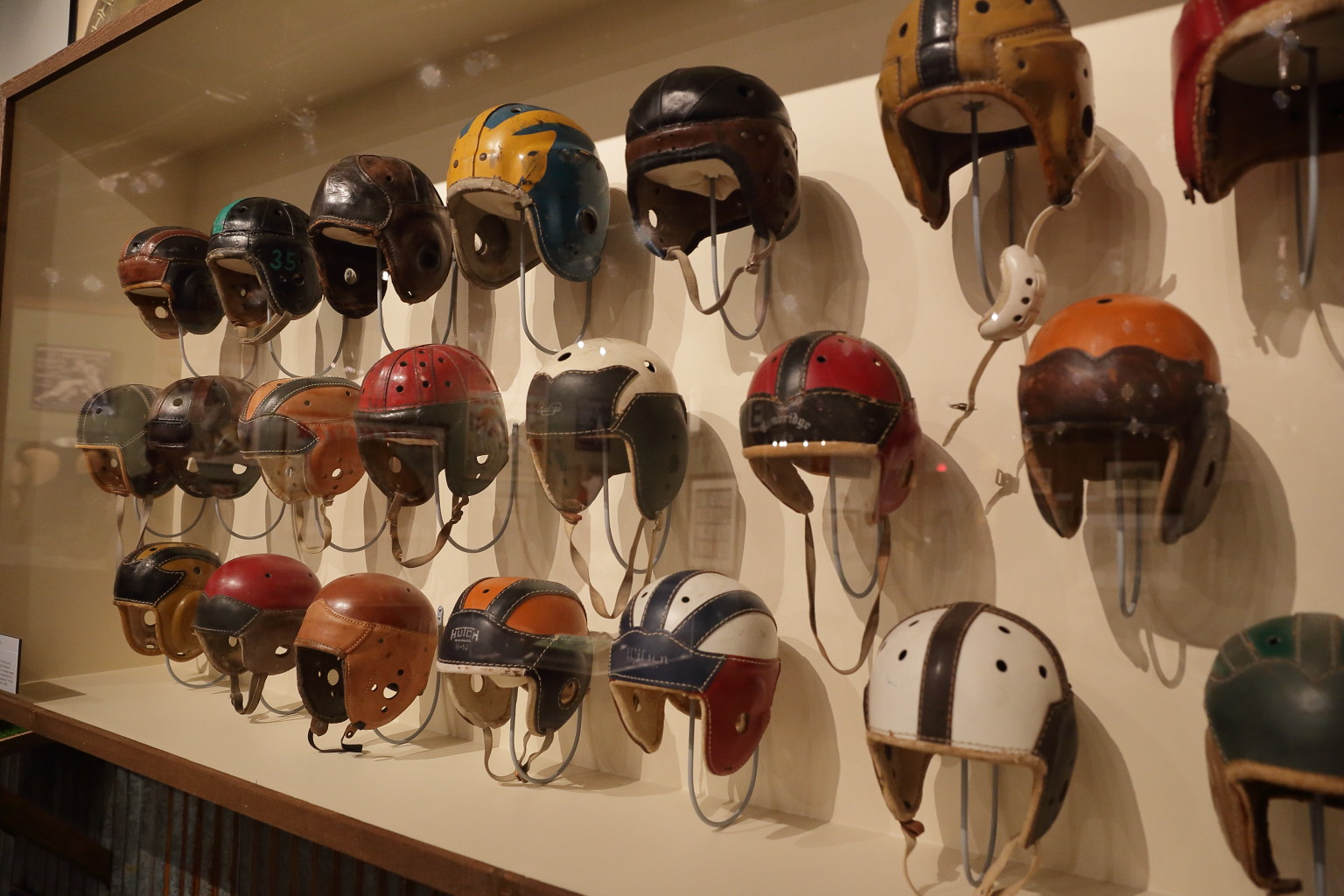The image showcases a white-inside, brown-wood outside display case housing 21 vintage-style football helmets, arranged in three rows. Each helmet varies in color and markings, resembling team representations, although no specific teams are identifiable except for one that resembles a Michigan Wolverine helmet. The helmets lack face masks and feature extended flaps for ear and head protection, giving them an antique appearance. Some of the notable color combinations include brown and black, blue and yellow, red and black, and red, white, and blue. The case stands against a gray slatted wall and has a nearly invisible glass front, more discernible on the left side with a slight reflection. A possible placard is partially visible at the bottom left but remains out of view.